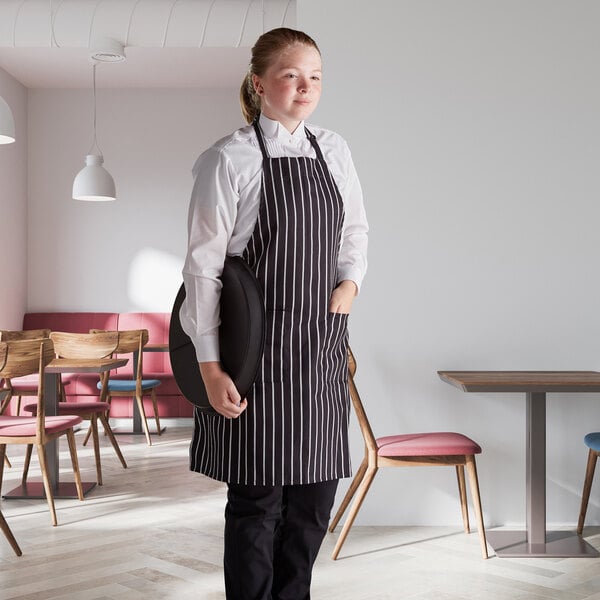In this image, a young woman, likely a server, stands centered in the frame. She is attired in a crisp white button-down shirt paired with black pants. Over her shirt, she wears a black apron featuring white stripes, with her left arm casually slipped into its pocket. Her right hand holds a serving tray, which she keeps close to her body. The scene around her is minimally adorned, emphasizing its clean and modern aesthetic. A table with a red-seated wooden chair and a gray table with a matching base are visible, along with partial details of a blue chair leg. The background reveals more seating options, including a couch along the wall and an array of brown, red, and blue chairs. A white pendant lamp hangs from the ceiling, casting a soft light over the setting. The young woman, with her gaze directed downward, adds a contemplative touch to the serene ambiance of the image.